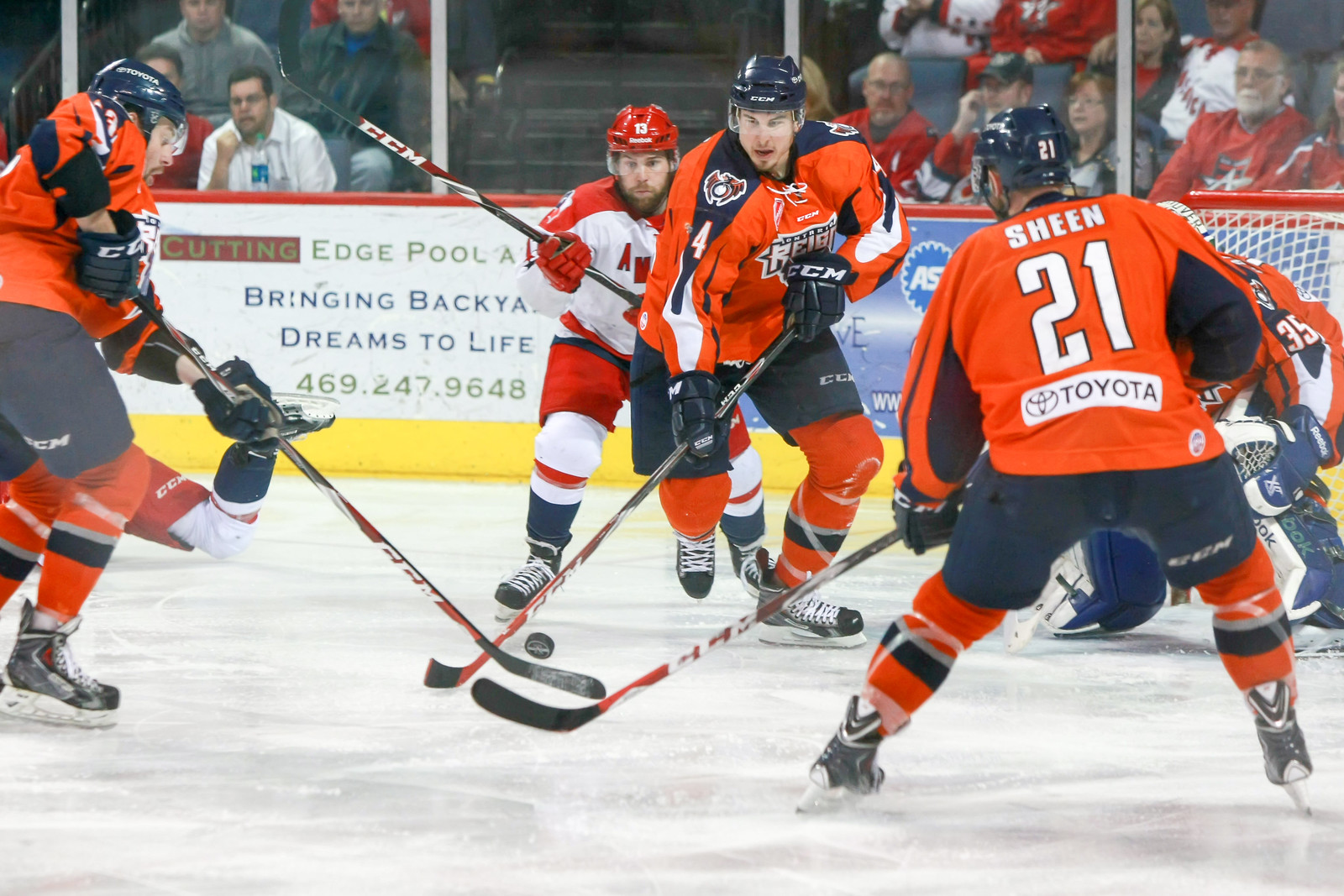This image captures an intense professional hockey game featuring two teams. Dominating the frame are players from the Ontario Reign, easily identifiable by their orange jerseys with navy blue shoulders, and black helmets. The player at the center, wearing the number 4 jersey, is actively pursuing the puck on the ice. Nearby, to the right, is his teammate, number 21, last name Sheen, and their sponsor, Toyota, is visibly emblazoned on their uniforms. Another teammate, number 35, and a fallen player, who is sliding on the ice face down with only their legs visible, can also be spotted. The opposing team, dressed in white jerseys with red shoulders and red helmets, has one prominent player in the frame slightly behind the central number 4 player. The game is being closely observed by a background crowd through the protective glass, capturing the excitement and energy of the scene. The presence of the Ontario Reign's goaltender indicates they are positioned defensively in their zone during this moment of the game.